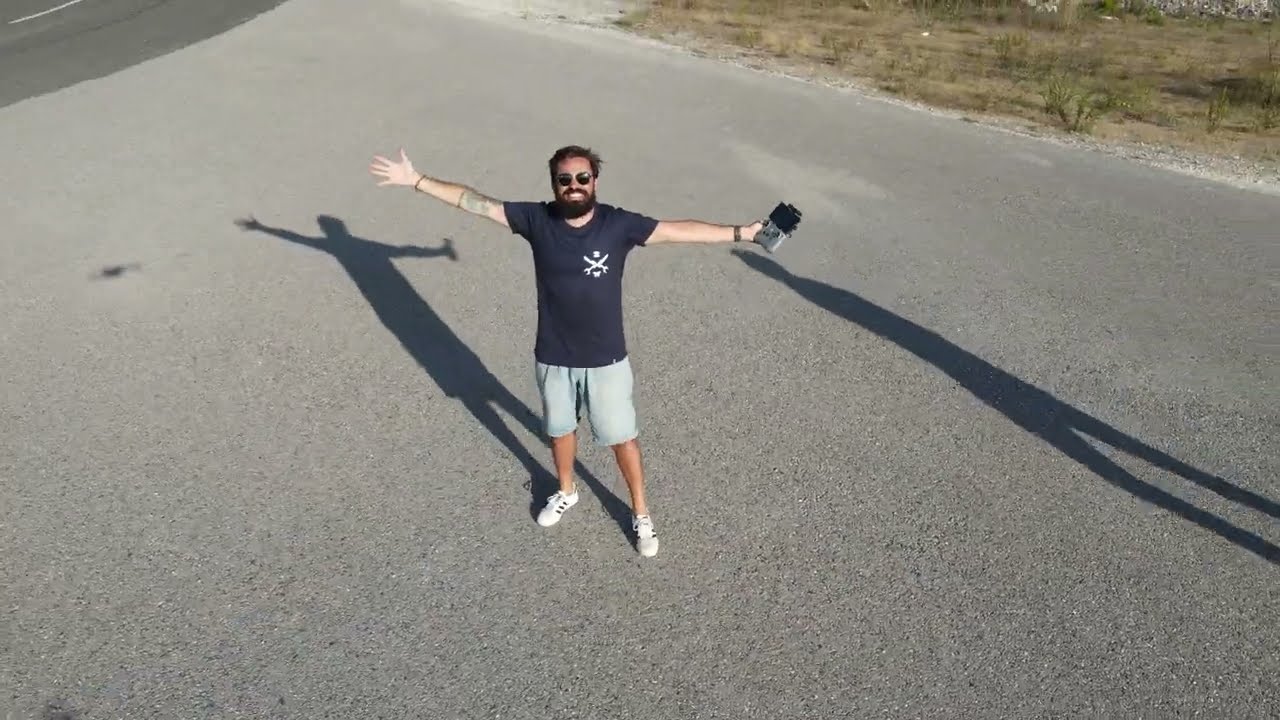The photograph features a bearded man with black hair, wearing dark sunglasses, and a big smile that reveals the white of his teeth. He stands on an open piece of asphalt with his arms outstretched. The man is dressed in a black t-shirt adorned with an emblem resembling a white cross made of swords where a pocket would typically be, gray shorts, and white tennis shoes. He wears a bracelet on his left wrist, which is holding a remote control, while his right wrist sports a wristwatch, and that hand is wide open. The scene behind him displays a desert landscape with brown dirt and scattered green bushes. A prominent shadow is cast behind him, and another shadow from an unseen figure appears in the bottom right corner of the image. In the upper left corner, the asphalt appears darker, suggesting a patch of different material.